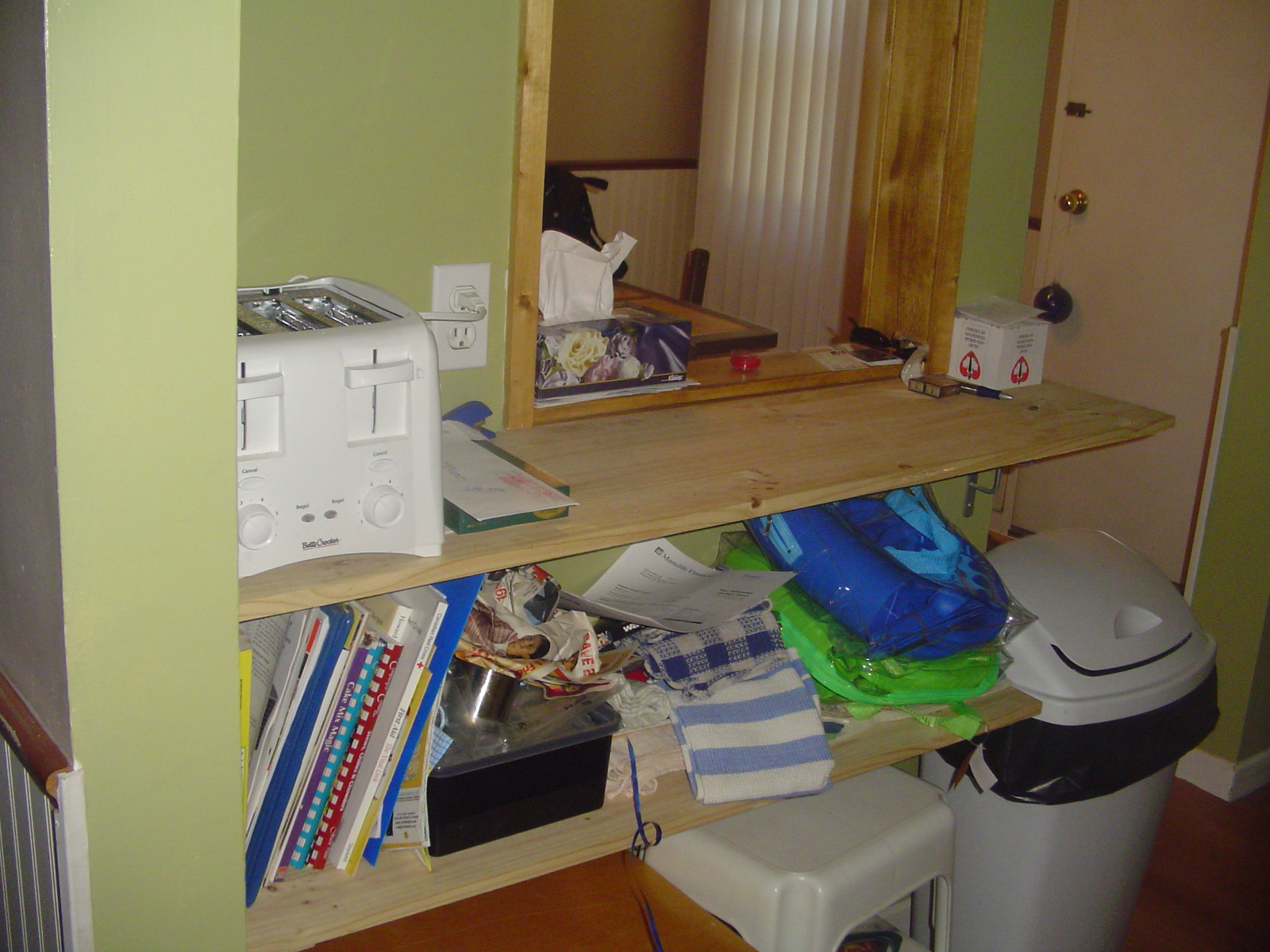In this indoor color photograph, we observe a room with pale green walls adorned with two horizontally-mounted wooden shelves. The top shelf displays a white toaster on the left side, featuring two push-down levers, chrome slots on top, and two white dials. The toaster is plugged into a white outlet via a white cord. Just beyond the toaster, there's a square hole in the wall, framed with thin wooden pieces. 

Beneath the top shelf, the lower shelf houses a collection of books and notebooks stacked vertically, leaning towards the right. Among these, a black plastic container is positioned alongside some blue and white dishcloths. The shelf also holds a fluorescent green item that appears to be a flattened backpack, topped with a blue object, possibly another backpack.

Below the second shelf sits a white square stool, and to the right of the shelving unit stands a tall white plastic garbage can with a lid, over which a black garbage bag is draped.